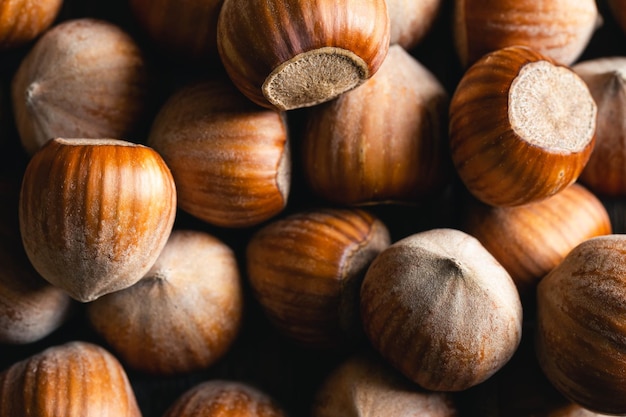A vibrant, color photograph showcases a substantial pile of hazelnuts, the image solely dedicated to these delicious nuts. At least a dozen hazelnuts fill the frame, each displaying their distinct, rounded bodies with flat tops that gracefully taper to a small point. The hazelnuts are clad in their natural, smooth brown shells, which exhibit a slight sheen in certain areas, adding texture and visual interest. The composition is entirely focused on the hazelnuts, devoid of any extraneous elements such as text, people, plants, buildings, or signs. The simplicity of the background enhances the rich, earthy tones of the nuts, making them the undeniable focal point of this meticulously detailed photograph.